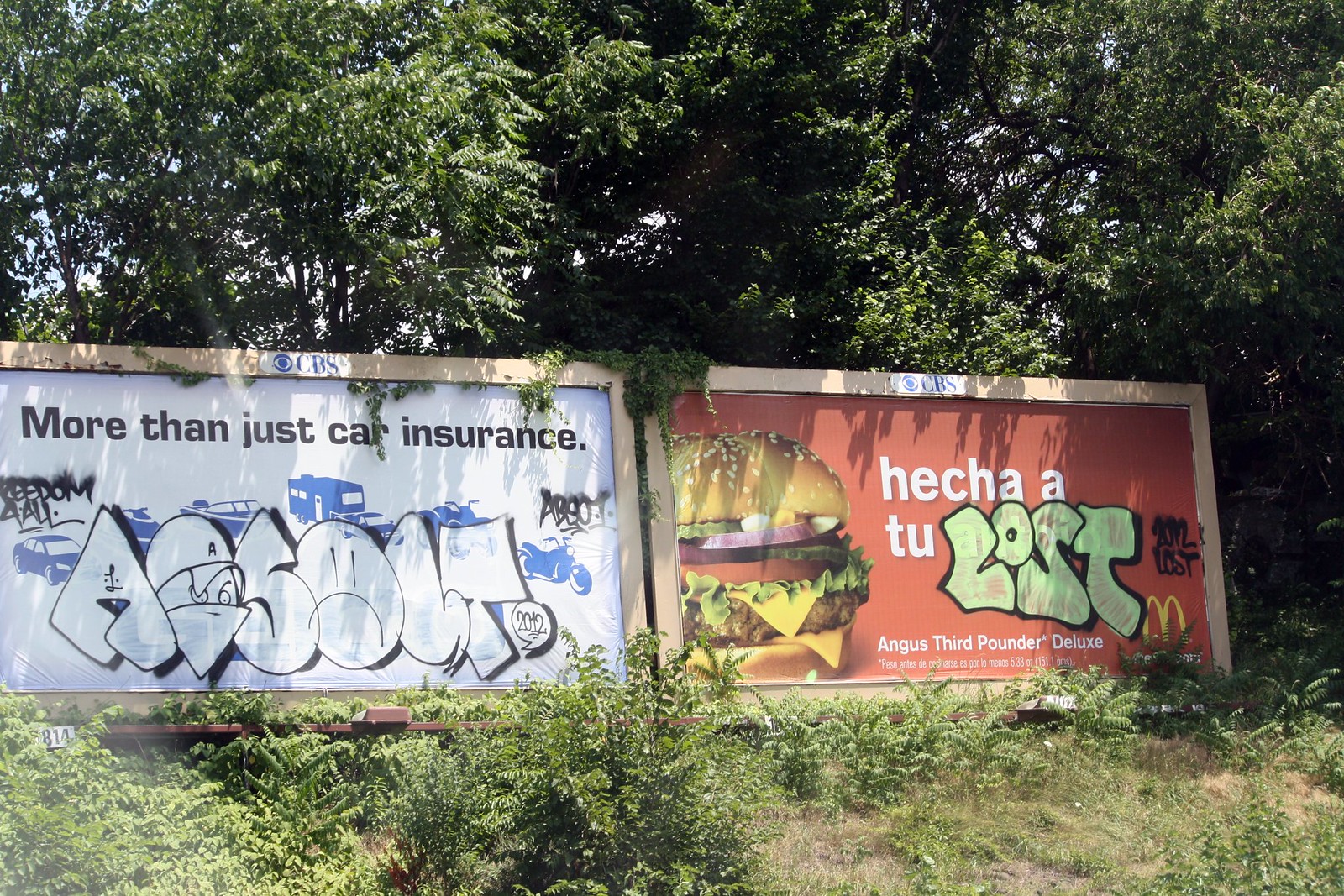The image depicts two adjacent billboards standing in the middle of a field overgrown with ferns and patchy grass. Overhead, leafy green trees extend their branches, providing a partial canopy. The billboard on the left displays the CBS logo at the top with the text "More than just car insurance" against a white background. The lower part of the billboard features blue silhouettes of various vehicles. This sign is heavily defaced with white and black graffiti. The adjoining billboard on the right advertises McDonald's Angus third-pounder deluxe. It has a vivid red background with a picture of the third-pounder burger in the left-hand corner and the McDonald's logo on the right. The promotional text is in white Spanish writing and the billboard is vandalized with graffiti that says "lost" in light green outlined in black.